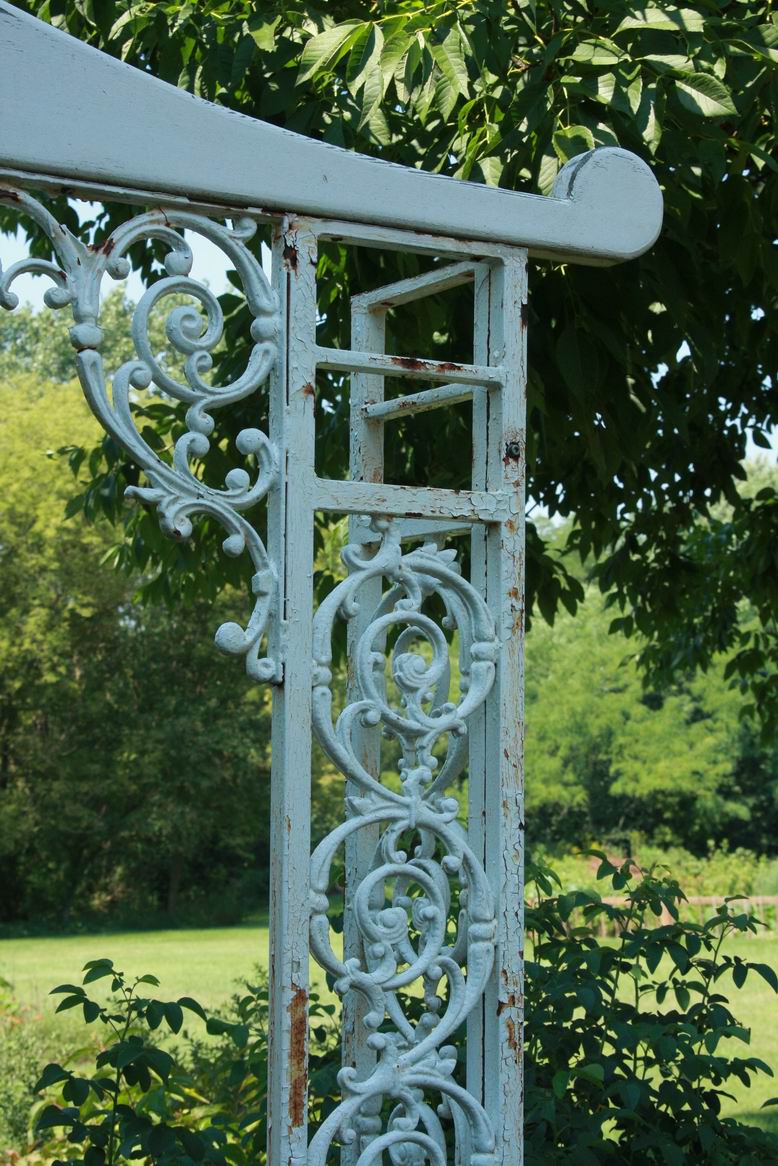The image captures a sunny day in a well-manicured garden, featuring an ornate metal archway structure that forms an entrance or gate. This archway, predominantly light blue but showing signs of age with patches of rust, is intricate in design, adorned with swirling vine patterns and circular, flower-like motifs. Constructed from welded square steel piping, it boasts a larger steel plaque-like design at the top, which angles down and swirls to the right. The right half of the archway, and part of the top, dominate the frame. Behind the structure, the vibrant green grass is neatly trimmed, with small bushes at the base giving way to larger shrubs and a tree overhanging the top right corner of the gate, creating a picturesque and serene garden setting.